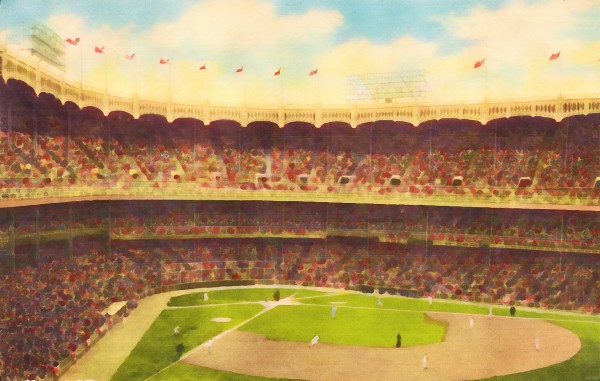This striking watercolor painting depicts a bustling baseball park from the left-hand side of the stadium, executed with impressive skill given the challenging medium. Against a backdrop of daytime skies with scattered clouds and patches of blue, the stadium's top is adorned with lighting structures and flagpoles flying red flags. Below, bunting-style wooden archways frame the steeply rising rows of bleacher seating filled with indistinct, smudged figures capturing the crowd's essence.

The green field below is meticulously detailed with a baseball diamond and painted lines. It appears the game has reached an intense moment, with bases loaded. The players, distinguished by their uniforms, are vivid yet impressionistically represented. The defense team, clad in white, is strategically positioned in the outfield, while the black-shirted players man the bases, poised to score. Interspersed, the referees are also visible, adding to the scene's authentic dynamism. Despite the medium's limitations, the painting captures a vibrant, immersive snapshot of a thrilling baseball game.